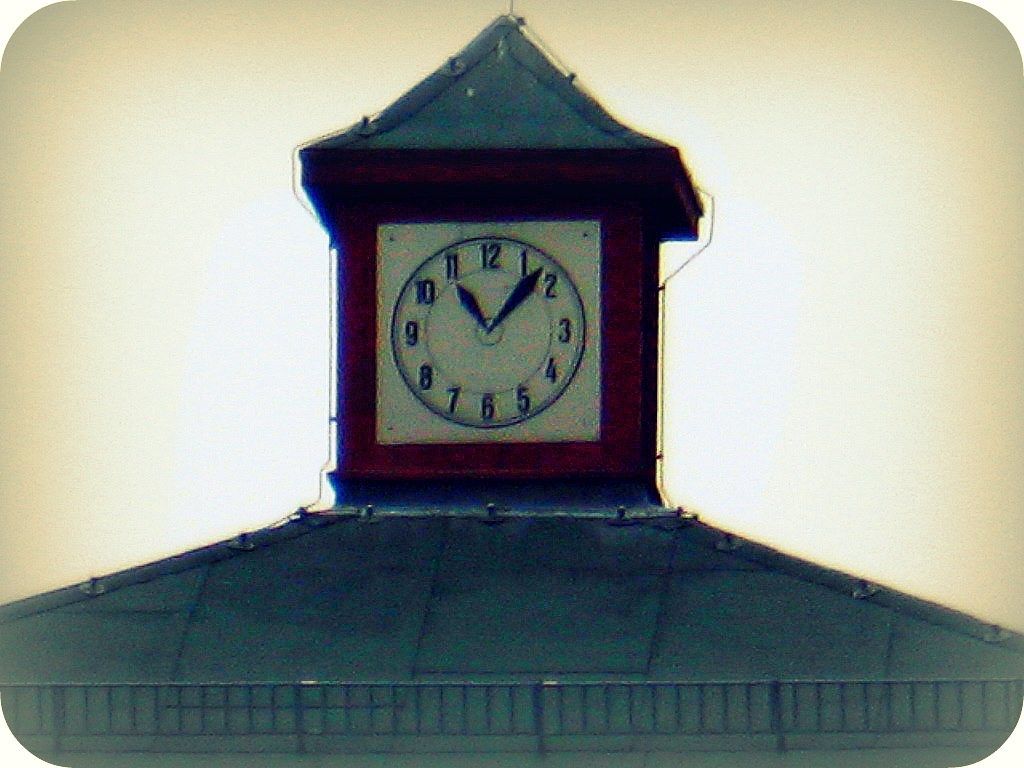The photograph, taken from outside, captures a detailed view of a clock mounted on the flat peak of a triangular-roofed building. The roof's apex, where one would expect a pointed finish, features instead a rectangular wooden housing for the clock, with a small triangular point crowning the clock’s top. This wooden casing, in a rich brown hue, frames a square clock face with a pristine white background. Black numerals clearly mark each hour, and matching black hour and minute hands indicate the time as approximately 11:08. The roof itself appears textured, possibly with paper or another material, and a metal railing stretches horizontally across the lower portion of the photograph, adding an additional element to the composition.